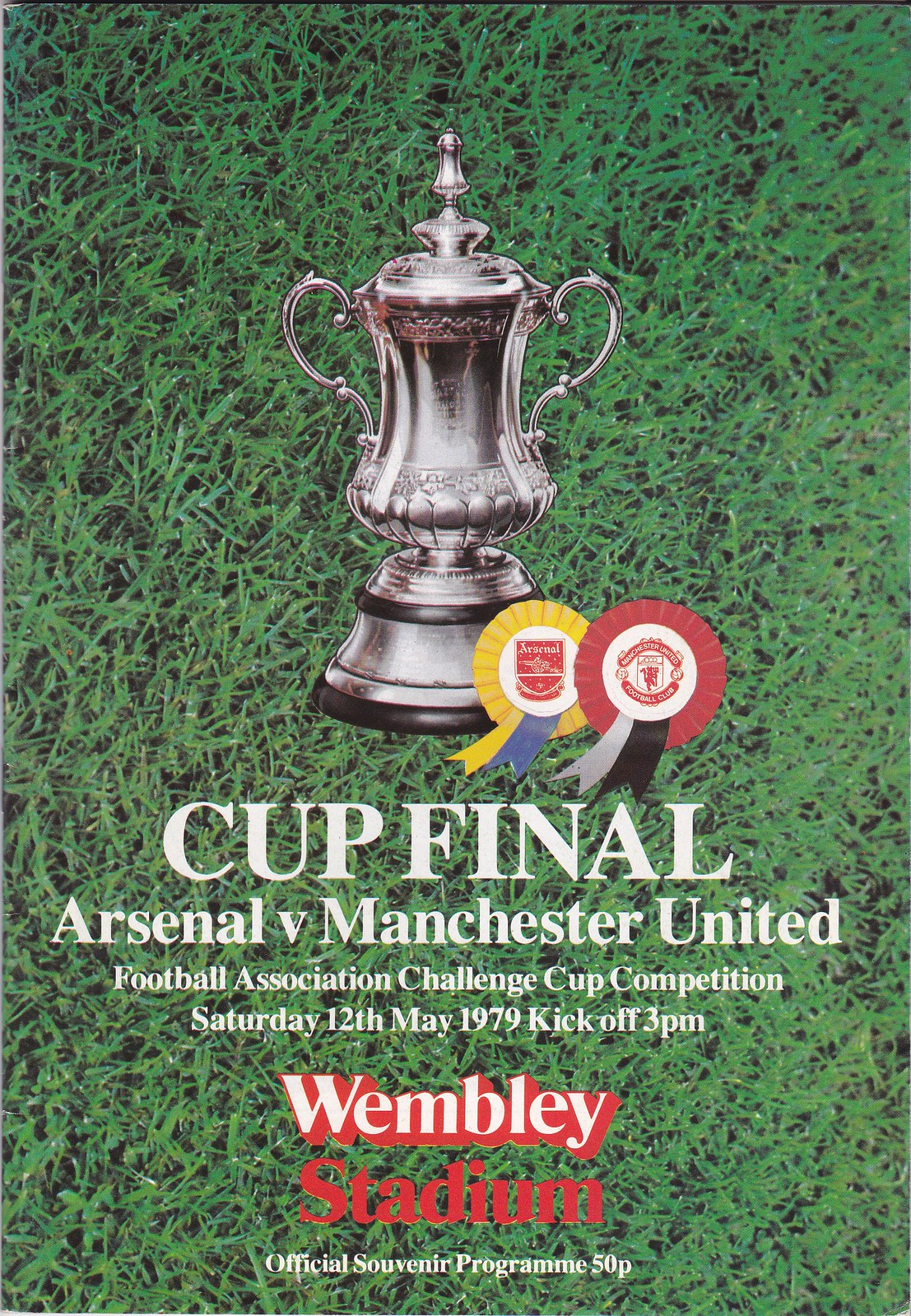This is a rectangular flyer with a vivid green grass background, depicting an English football program for a Cup Final. Dominating the center of the flyer is a silver trophy with two handles on either side and a lid. Accompanying the trophy are two ribbons: one is yellow with blue and red accents and a white center, while the other is red with silver and black accents and a white center. Prominently displayed above the trophy are large white letters reading "Cup Final." Below, the flyer details the match: "Arsenal vs. Manchester United, Football Association Challenge Cup Competition." Additional information includes the date and time: "Saturday, 12 May 1979, kickoff, 3 p.m.," and the location: "Wembley Stadium." At the bottom, red letters on a white background state, "Official Souvenir Program, 50 pence." The fonts vary in size from very large to very small, mostly in white against the green background, with Wembley Stadium highlighted in both white and red. The overall color scheme prominently features green, yellow, blue, red, silver, black, and white.